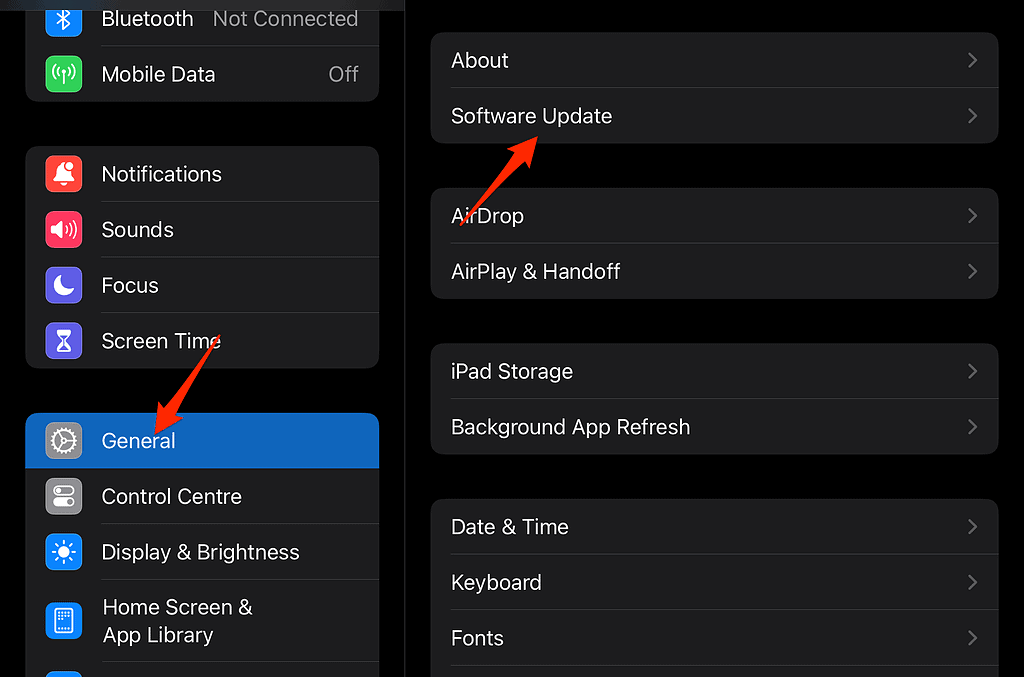A detailed caption for the image:

---

The image depicts a settings page on an Apple device, presented in dark mode with a black background and dark gray tabs, creating a sleek and modern aesthetic.

**Top Left Corner:**
- **Bluetooth:** Displayed with the iconic blue Bluetooth symbol next to the white text "Bluetooth," followed by "Not Connected" in gray text.
- **Mobile Data:** Represented by a green logo and gray text.

**Notification Section:**
- A red and white bell icon indicates the notification settings, with the text "Notifications" in white.

**Sound Section:**
- A pink and white icon symbolizes sound settings, labeled "Sounds" alongside it.

**Focus Section:**
- Two purple icons are shown:
  - The first features a white crescent moon with "Focus" written beside it.
  - The second shows a white hourglass icon with the label "Screen Time."

**General Settings:**
- An actively selected button is labeled "General," accompanied by a gray gear icon.
- A red arrow, presumably added through image editing, points to the "General" section.

**Control Center:**
- A subsequent gray icon represents the Control Center settings.

**Display and Brightness:**
- A blue sun-like icon labeled "Display & Brightness."

**Home Screen and App Library:**
- Immediately below is another blue icon representing a phone screen, labeled "Home Screen & App Library," though partially cut off.

**Right Side of the Image:**
This side contains several clickable options set within dark gray boxes with white text:
- **About:** Located at the top.
- **Software Update:** Marked with an edited red arrow pointing toward it.
- **Additional Options Include:**
  - AirDrop
  - AirPlay & Handoff
  - iPad Storage
  - Background App Refresh
  - Date & Time
  - Keyboard
  - Fonts

The image conveys a clear and organized overview of various settings available on the device.